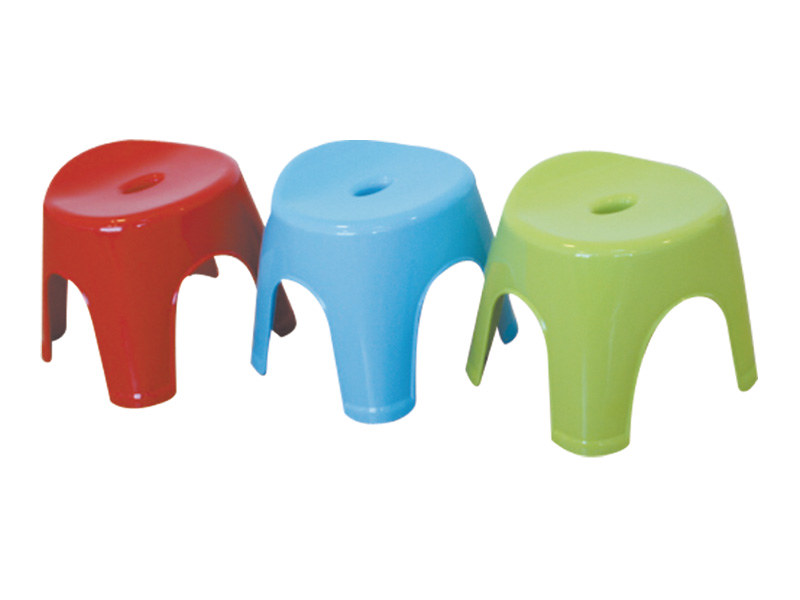This image is a product photo showcasing three identical children's stools, photographed against a plain white background to emphasize their vivid colors and shiny plastic material. The stools, molded from a single piece of plastic, are arranged in a straight line with slight interlocking of their legs, creating a clean, organized appearance. Each stool features a slightly curved seat with an oval hole in the center for ease of carrying, and they rise to about a foot and a half in height. The stool on the left is a bright cherry red, the one in the center is sky blue, and the stool on the right is an avocado green. All three stools are new, reflecting light off their unblemished surfaces, suggesting they have never been used. The uniform design includes slightly curved, four-legged bases with arch-like gaps in between, adding both aesthetic appeal and stability.